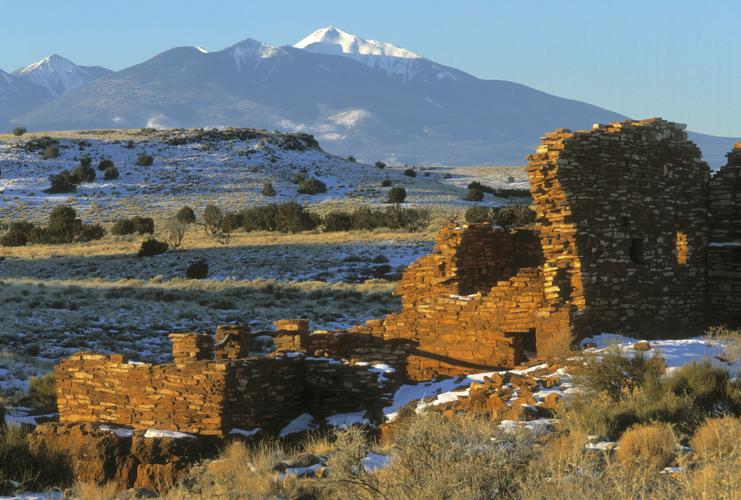The photograph captures a serene nature scene, showcasing the rugged beauty of a snowy plains landscape at the foot of the Rockies. In the foreground stand the ruins of ancient stone structures, possibly remnants of Native American dwellings, characterized by partially standing brick walls. These ruins, composed of brown and white bricks, suggest a timeworn history as they lie in disrepair. The ground around these structures is a patchwork of snow cover interspersed with unkempt, tan grasses and clusters of green bushes. To the left, a gentle hill slopes upward, leading the eye toward the background where majestic mountains rise, their peaks capped with glistening white snow. The sky above is a bright, light blue, adding to the tranquility of this wild, untamed landscape.